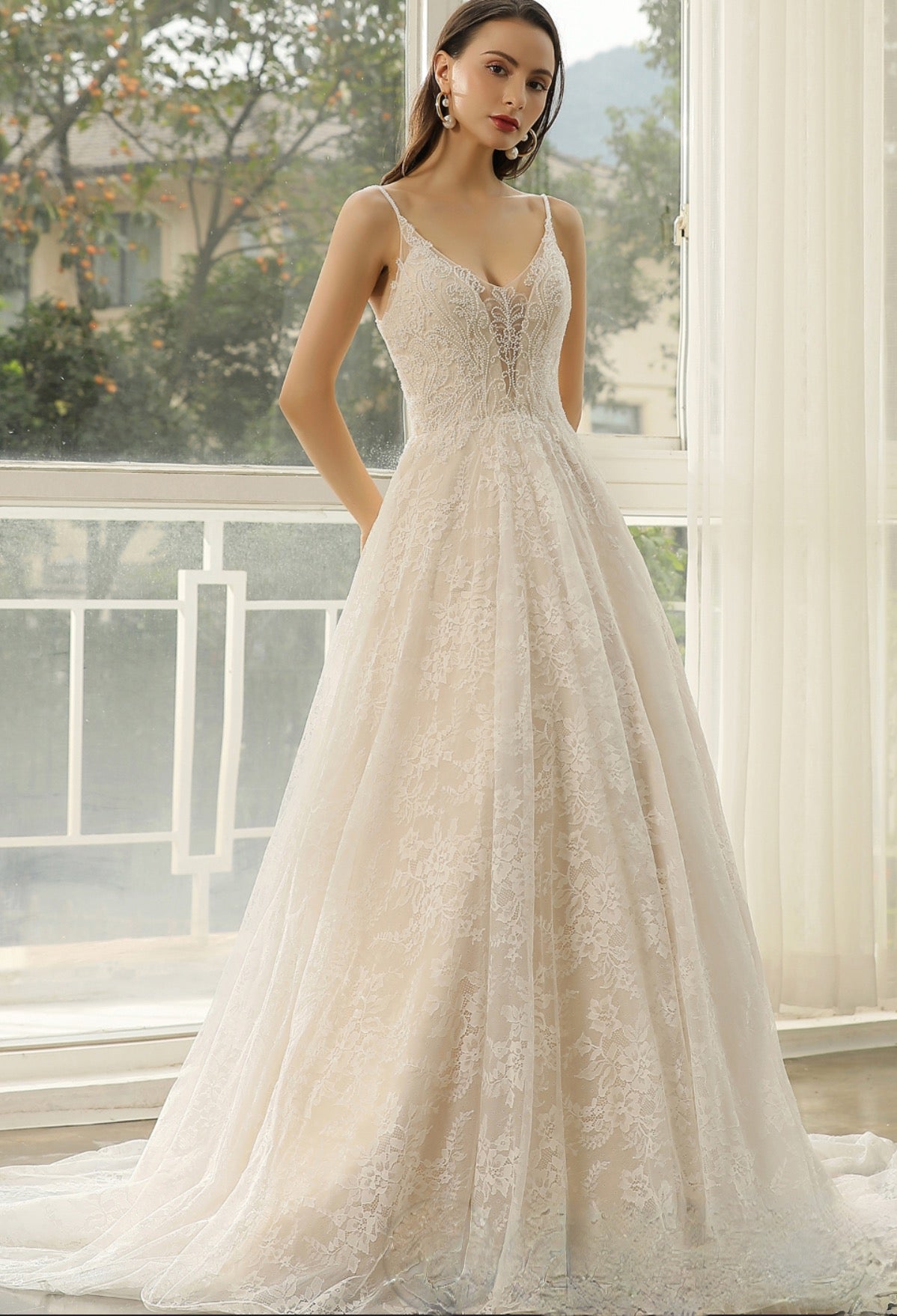The image features a stunning young woman, possibly computer-generated, standing gracefully in an elaborate, flowing white gown that resembles a wedding dress. The dress is exquisitely lace-adorned with an outer sheer layer, creating a delicate and elegant appearance. She has long, dark hair and is wearing hoop earrings with pearls dangling from them. Her makeup is stylish, featuring evening wear makeup with bold red lipstick. The dress is sleeveless with spaghetti straps and a gently rounded low-cut neckline, fitting her very thin, fair-skinned figure beautifully. She stands poised, with her arms behind her back, directly facing the camera in a sophisticated pose. Behind her, a window reveals the outdoors, where a balcony with drapes matching the fabric and color of her gown is visible. Through the window, trees adorned with citrus fruits and light-colored buildings further enhance the soft, whimsical ambiance of the setting. The floor appears to be crafted from beige marble, adding to the upscale and formal atmosphere of the scene.